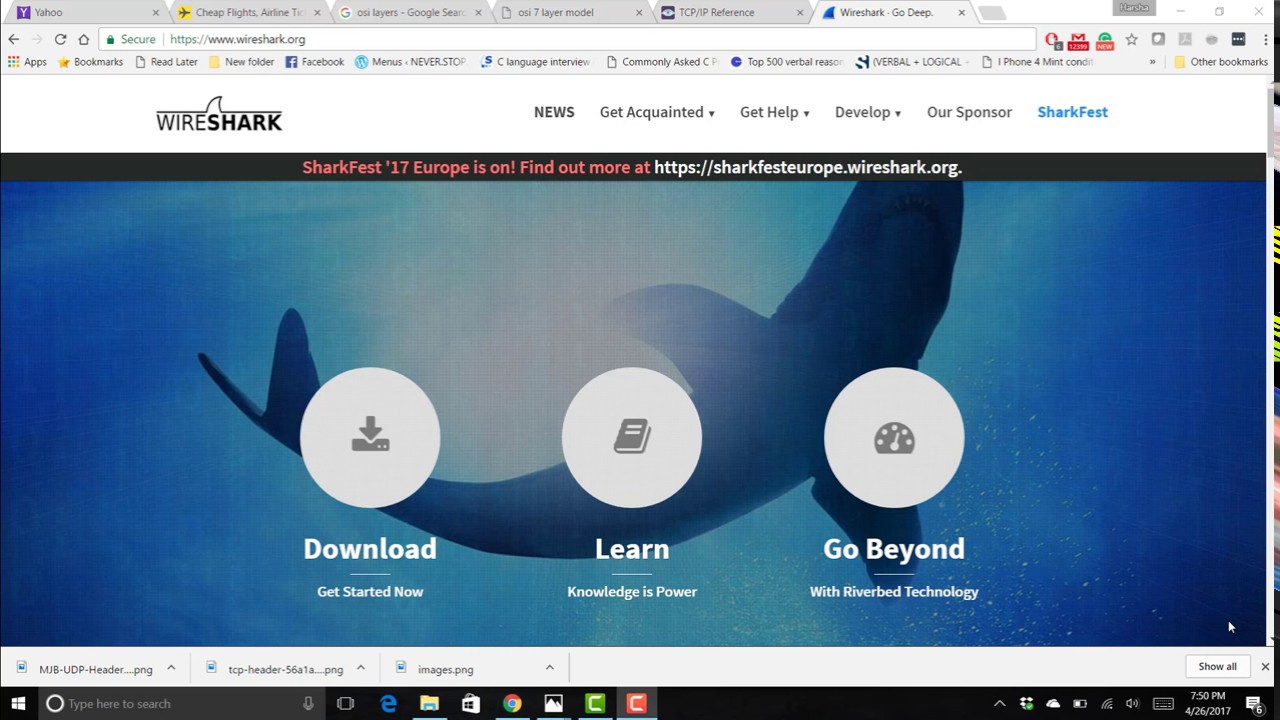The image is a screenshot of a website, specifically a page from Wireshark's official site. At the top of the browser window are six tabs: 

1. Yahoo
2. Cheap Flights, Airlines,
3. Aussie Layers
4. Google Search
5. Aussie Seven Layer Model, 
6. TCP/IP Reference
7. Wireshark GoDeep (highlighted in light blue).

Below the tabs is an address bar displaying the URL: https://www.wireshark.org. 

To the right of the address bar sits an email icon with an astonishing count of 12,000 unread emails, accompanied by a red circle with a white hand symbol, a green circle with a white "G," a star, and three more icons.

On the left side of the browser, there's a vertical list including:
- Apps
- Bookmarks
- Read Later
- New Folder
- Facebook
- Menus Never Stop
- Language Interview
- Commonly Asked Questions
- Top 500
- Verbal Reasons
- Verbal Plus Logic
- iPhone 4 Mint Condition

To the right of these bookmarks, it says "Other Bookmarks."

In the main content area of the website, at the top left, it reads "Wireshark" with a shark fin logo. Below this are several navigation links:
- News
- Get Acquainted
- Get Help
- Develop
- Sponsors
- Shark Fest

Further down, there's a large, engaging image of a shark swimming underwater, oriented head-up towards the right and tail towards the left of the image.

Above this oceanic scene, the URL https://www.wireshark.org is once again displayed. Additionally, there are three circular icons with descriptive labels:
- A download icon labeled "Download"
- A book icon labeled "Learn" with the tagline "Knowledge is power"
- A clock or timer icon labeled "Go Beyond."

Overall, the page appears to be richly detailed, helping users navigate various resources and information related to networking protocols, specifically through Wireshark tools and knowledge.